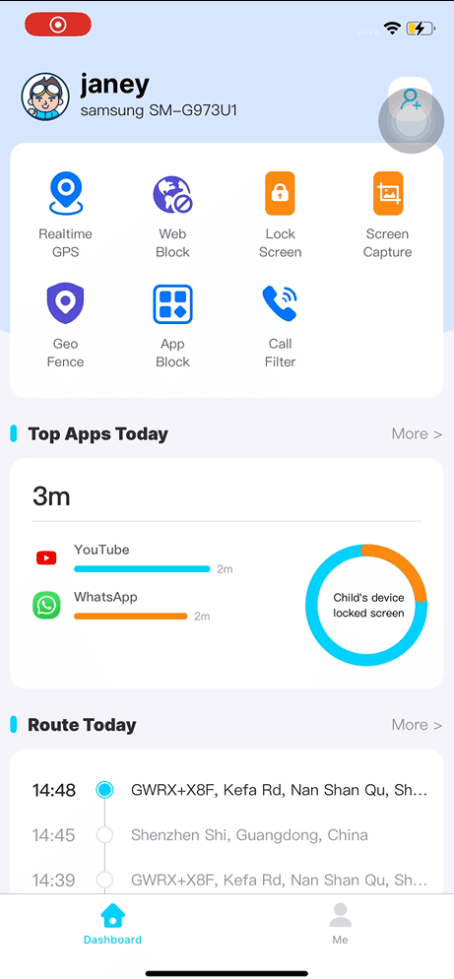This image is a detailed screenshot captured on a smartphone, seemingly from a screen recording. In the upper left corner, there is a long oval icon that is red, containing a white target symbol in the center, indicating an ongoing recording. In the upper right corner, there are standard phone indicators including a Wi-Fi icon and a battery icon that shows a bit of yellow and a lightning bolt, suggesting the phone is charging.

The screenshot is primarily divided into three distinct sections with a white foreground on a light blue background. 

At the top section, an avatar of a cartoon person wearing goggles on their forehead is visible next to the name "Janie" written in black text. Below this, it reads "Samsung SM-G973UI," indicating the device model.

The first section consists of seven icons labeled as follows: Real-time GPS, Web Block, Lock Screen, Screen Capture, Geofence, App Block, and Call Filter. 

The second section is titled "Top Apps Today." It features text in black, showing "3M." Underneath are icons for various apps: the YouTube logo with the name "YouTube" and a blue progress bar indicating "two minutes," followed by the WhatsApp icon and the name "WhatsApp" with an orange icon also indicating "two minutes." On the right side of this section, a blue circle with a small orange segment reads "Child's device locked screen."

The third and final section is titled "Root Today."

The entire layout seems to be part of a parental control or device monitoring application, as inferred from the icons and section titles.